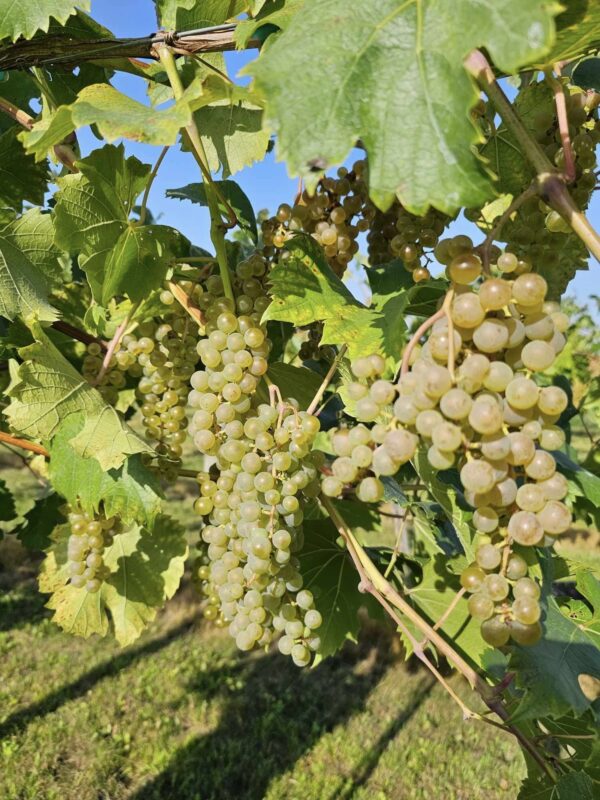This close-up, daytime color photo captures lush green grapes hanging in multiple large bunches from a thick brown vine. The main vine stretches horizontally across the top of the image, with numerous smaller vine branches extending downward, intertwining around the grapes and headed toward the grassy ground below. The bright green leaves are broad and abundant, providing a vibrant backdrop to the clusters of grapes, which range in size from small to ripe and plump. The sunny sky, vivid and cloudless, peeks through the top of the frame, highlighting the healthy, unfallen grapes. Additionally, a line that appears to tie the grapevine securely runs beneath the main vine, and a shadow of the person taking the photo is visible on the sparse grassy ground, where patches of dirt are interspersed. The entire scene suggests a thriving grapevine, captured in the midst of a sun-drenched day.